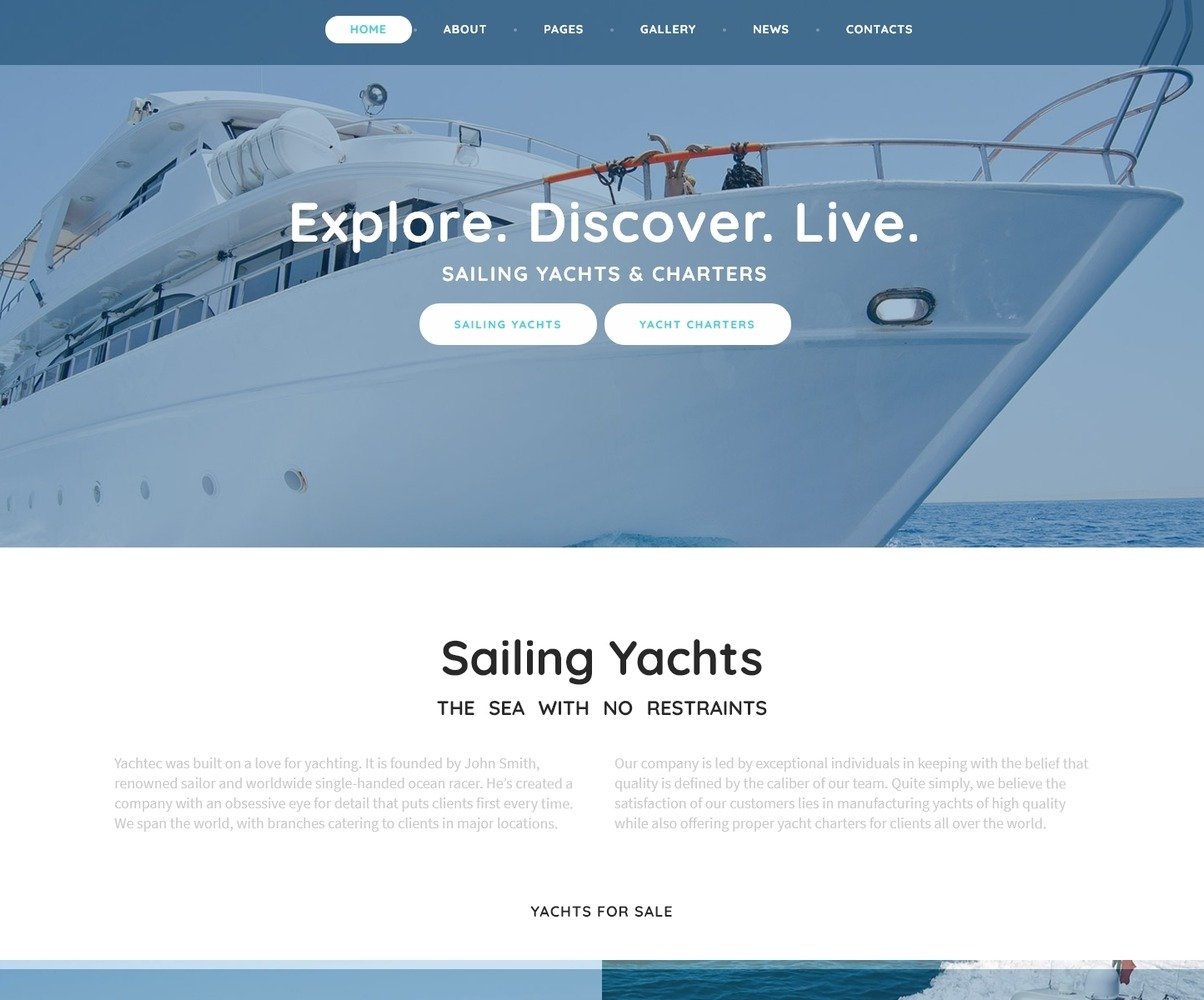At the very top, a dark blue banner runs horizontally across the width of the webpage. It contains various menu options such as Home, About, Pages, Gallery, News, and Contacts. Beneath this banner, the layout transitions to a lighter blue section that prominently displays an image of a sleek yacht. The yacht's deck features what appears to be an anchor positioned on the railing. The background showcases a serene blend of blue sky and vast blue waters.

Superimposed on this picturesque scene is the phrase "Explore, Discover, Live, Sailing Yachts and Charters," inscribed in crisp white text. Below this, the title "Sailing Yachts" is displayed in bold blue letters on a white background, accompanied by "Yacht Charters" also in blue on white.

Further down, a caption in black reads, "Sailing Yachts—The sea with no restraints," introducing a white-textured section that contains several paragraphs detailing the company's history. Founded by the renowned sailor John Smith, the company is elaborately profiled.

Toward the bottom of the page, there is an announcement in darker letters promoting "Yachts for Sale." Finally, the webpage concludes with a dark blue banner at the very bottom, mimicking the look of deep water, tying the visual theme together.